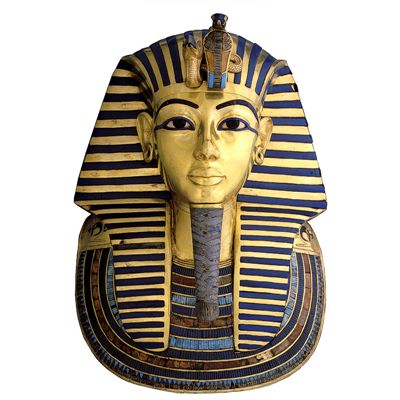This image showcases the iconic ancient funeral mask of King Tutankhamun, renowned worldwide. The bust is adorned with the Pharaoh's distinctive striped head covering, made of alternating bands of navy blue and gold, which encircle the entire face and reveal the ears. The neutral-expressioned face, made of bold gold, navy blue, and azure details, is meticulously symmetrical, with open eyes and a closed mouth accentuated by traditional Egyptian makeup. Prominently displayed on the forehead are two emblems—a pair of serpents crafted in gold and black, with hints of blue. Below the face, the long, intricately wrapped beard extends downward, its design composed of series of thin strips, while the neck is encircled by an elaborate multi-colored collar, consisting of layers in silver, navy, brown, and varying shades of blue, all highlighted by gold trim. The image is set against a plain white background, drawing all focus to the ornate craftsmanship of the Pharaoh's mask.